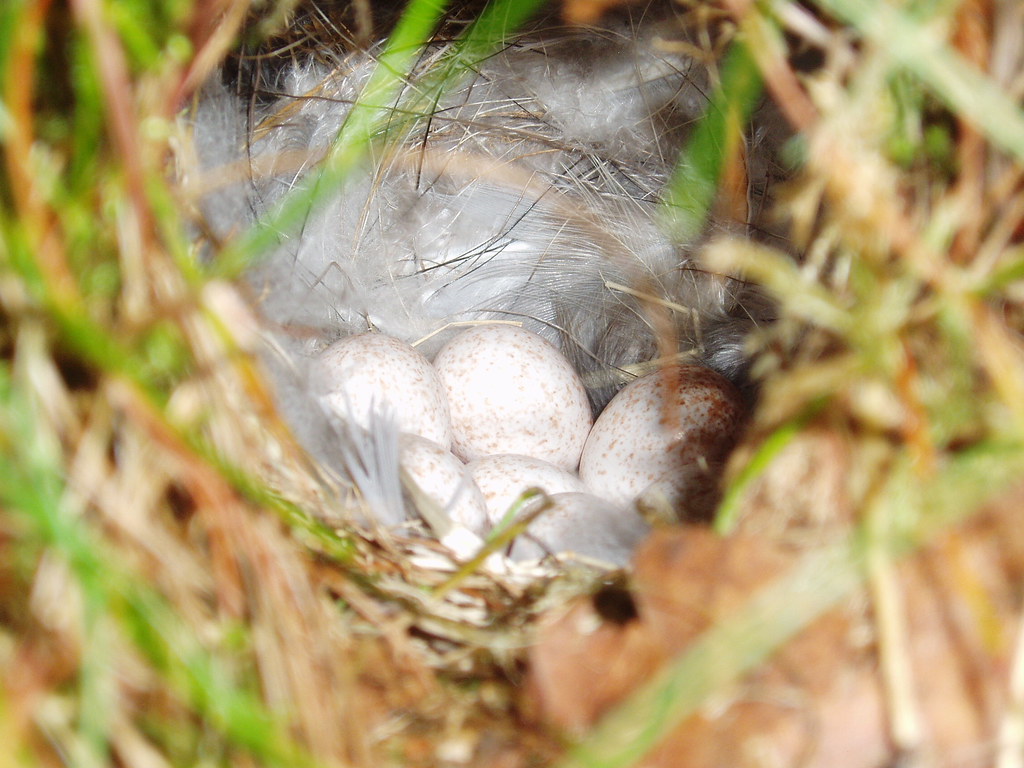This close-up photograph captures an intricately constructed bird's nest situated slightly above the center of the horizontal frame. The nest cradles six white eggs speckled with brown, nestled closely together. It's made up of a delicate bed of white and brown feathers, interwoven with green and brown strands of grass and an occasional brown leaf, creating a cozy, cave-like structure. The surrounding area, comprising blurry green and beige grass, frames the nest, drawing the viewer's attention to the detailed and brightly focused nest and its precious contents. The soft focus on the grass and other elements in the foreground further emphasizes the nest and the eggs as the main subjects of the image.